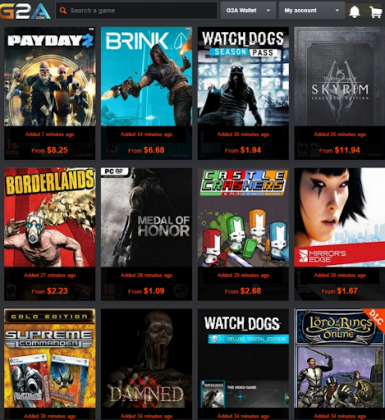The image features a web interface set against a gray background. Prominently displayed is the "G2A" logo, with the letters "G" in orange, "2" in white, and "A" in blue. Below the logo is a search box accompanied by an orange magnifying glass icon. There are two gray rectangles incorporated into the design, as well as options for navigating to the "G2A Wishlist," "My Account," notifications (indicated by a bell icon), and a shopping cart icon. 

A list of various game titles is presented, including:
- "Payday 2," where the "2" is colored blue,
- "Brink," displayed in white,
- "Watch Dogs Season Pass," with "Season" in white on a blue rectangle and "Pass" in black on a white rectangle,
- "Skyrim," spelled as "s-k-y-r-i-m" in white,
- "Borderlands," in a standard font,
- "Medal of Honor," likewise in a standard font,
- "Castle Crashers,"
- "Mirror's Edge,"
- "Supreme Commander,"
- "Down,"
- "Watch Dogs," (appears again),
- "Lord of the Rings Online."

The overall layout is intuitive, with a clean and organized aesthetic that groups navigational elements and game titles effectively.